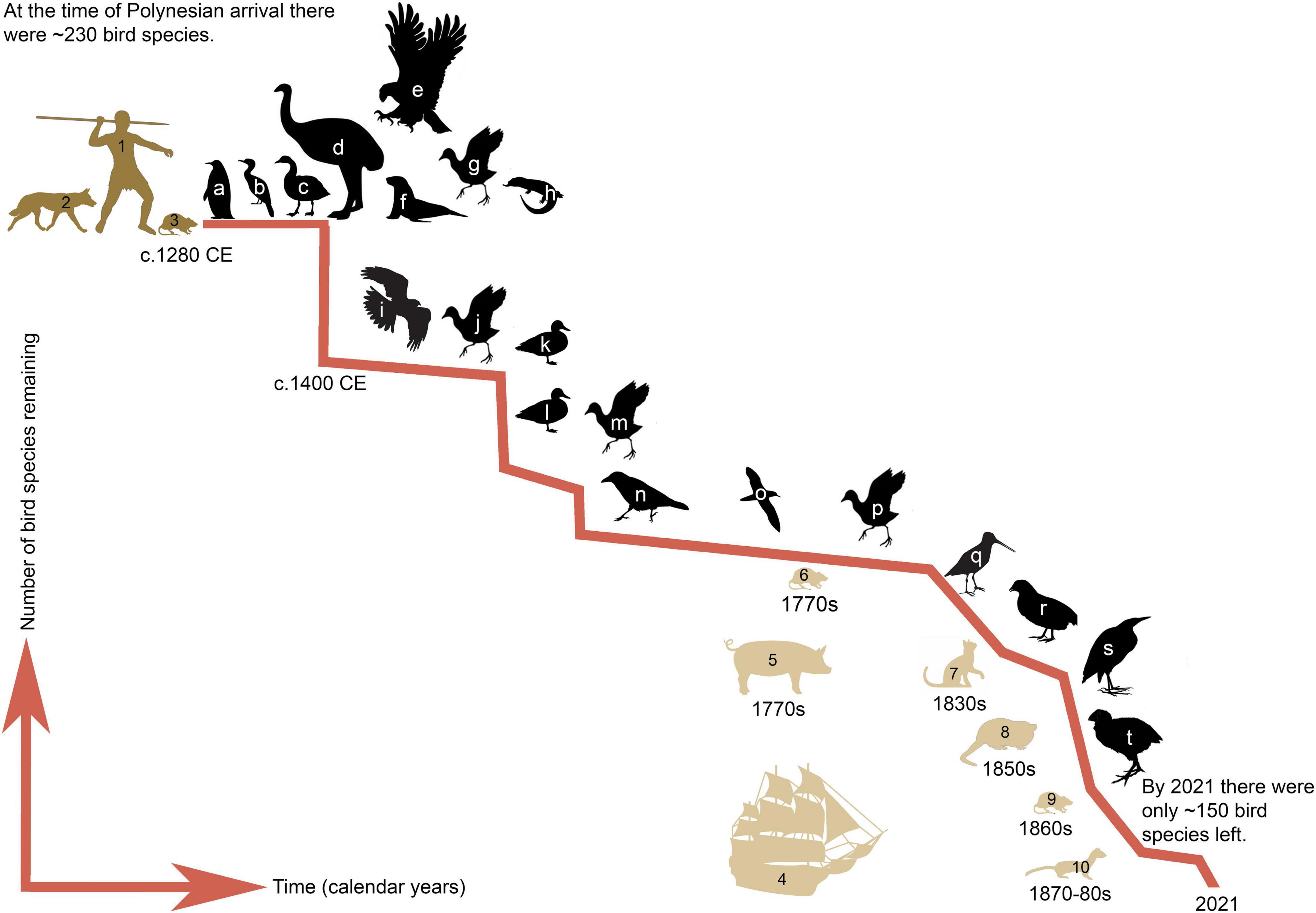This diagram charts the decline of bird species from the time of Polynesian arrival around 1280 CE to 2021. The y-axis represents the number of bird species, and the x-axis denotes time/calendar years. In the top left, there is a figure of a man holding a sphere or spear, accompanied by a dog/wolf labeled with the number "2," and a rodent labeled with the number "3." A red line descends diagonally from the top left to the bottom right of the chart, symbolizing the decreasing number of bird species. Along this line, silhouettes of various birds labeled from A to T, such as penguins, ducks, ostriches, eagles, and flamingos, illustrate different species over time. Beneath the line, closer to the bottom right, tan silhouettes of other animals and a ship appear, marked with corresponding letters and years. Text at the top left indicates that around 1280 CE, there were about 230 bird species, while the bottom right notes a reduction to approximately 150 bird species by 2021. Arrows on the left and right sides of the diagram label the axes as the "number of bird species remaining" and "time and calendar years," respectively.